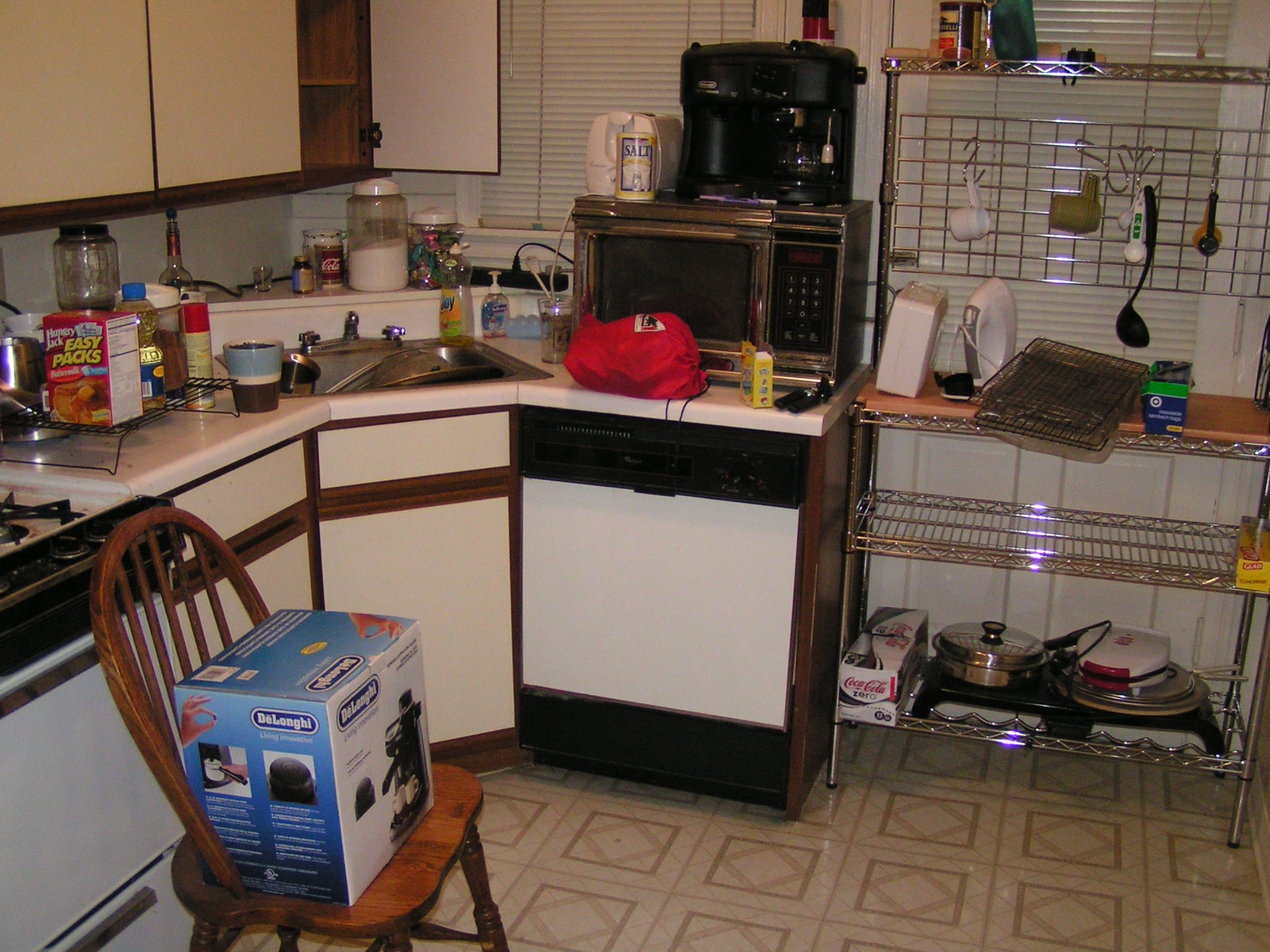The photograph showcases a neatly organized kitchen with a rectangular orientation, emphasizing its width. The floor features an intricate tile design, with each white square tile containing a smaller brown square at its center, which in turn has a brown diamond pattern inside.

On the right side of the image, a stainless steel storage shelf system stands prominently. The bottom shelf is packed with various cooking utensils, electronic cooking devices, and a white box of Coca-Cola. The middle shelf holds a single yellow rectangular box of plastic wrap, while the top shelf supports a brown mat along with assorted cookware, an iron, and a blue and green box of aluminum foil.

Above these shelves, a grated rack spans the top of the storage unit, equipped with stainless steel hooks carrying an array of cooking utensils, including measuring cups, a ladle, and measuring spoons. The kitchen's countertops are a clean white, paired with tan and brown cabinetry, contributing to a cohesive and functional kitchen space.